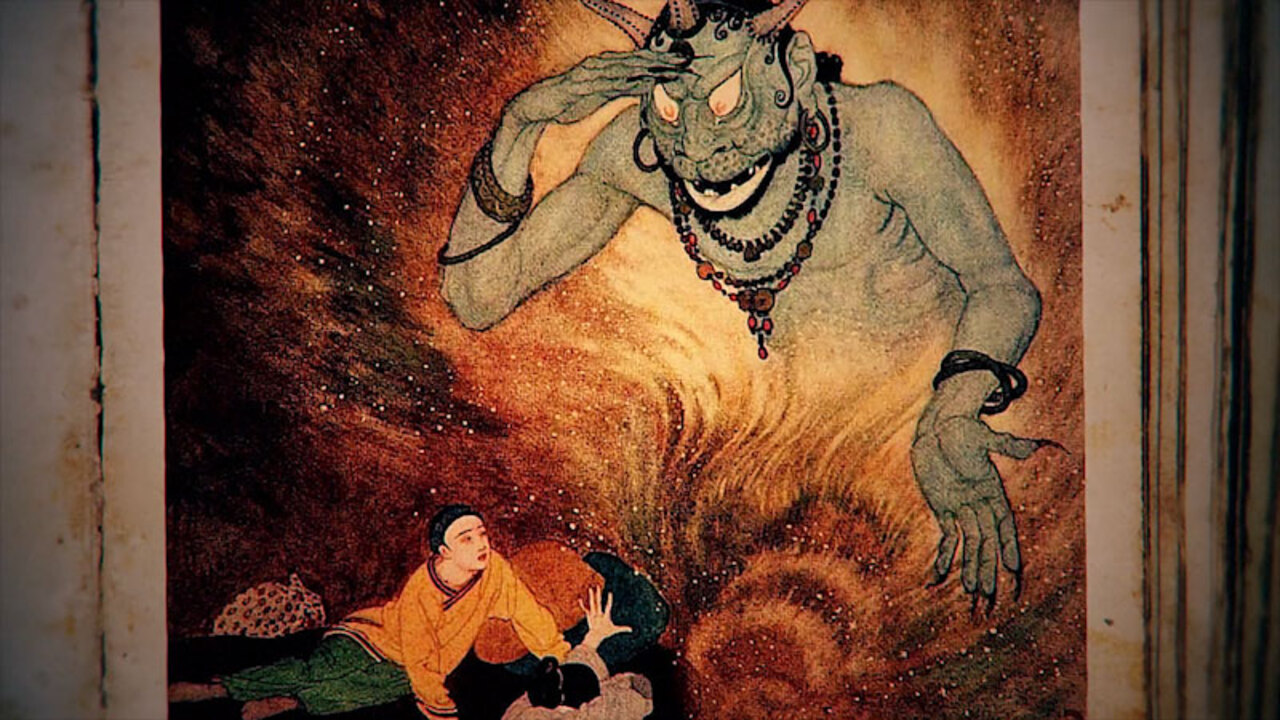The image appears to be a photograph of an old, possibly molded, vertical rectangular painting or mural, with visible frames on the sides but not on the top or bottom. The artwork vibrantly depicts a menacing demon emerging from flames in the upper right section. The demon is humanoid from the waist up, richly detailed with green skin, horns, evil-shaped eyes, and a mouth full of teeth. It is adorned with necklaces, earrings, and multiple bracelets, and it has long fingers ending in sharp claws. Below, on the lower left side, a woman—possibly Oriental, dressed in an orange top and black bottom—lays down, one hand raised as if trying to hold back the demon. Her closed eyes suggest reluctance or perhaps exhaustion from confronting the demonic presence. An additional hand, which appears out of place, raises ambiguity about another potential figure partially cropped out. The painting’s vibrant colors contrast starkly with the dirty, possibly dusty or moldy, surfaces surrounding it, adding an eerie ambiance as if highlighting the age and mystical essence of the depicted scene.